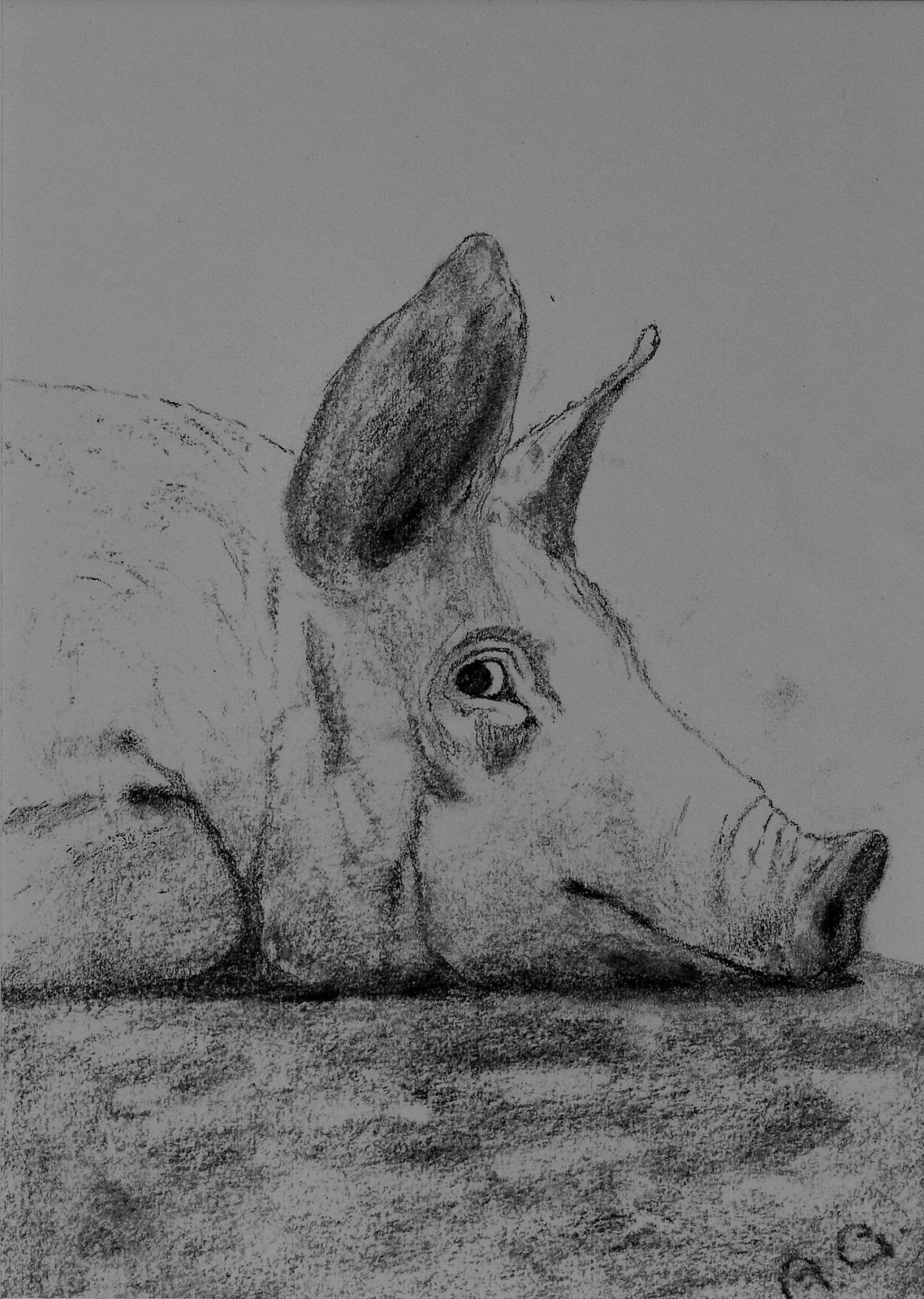This artwork, seemingly created with either charcoal or pencil, depicts a lifelike and detailed drawing of a pig lying on the ground. The illustration focuses on the pig from its forward shoulders to its snout, with its body oriented to the right. The pig's head rests on the ground, and its right eye is particularly striking, gazing directly at the viewer with an almost human-like expression. The pig's ears stand upright and alert, adding a sense of attentiveness despite its prone position. The artist has skillfully shaded the ground beneath the pig, enhancing the realism of the scene. The background is left intentionally blank, devoid of any extraneous details, which draws all attention to the pig itself. In the lower right-hand corner of the piece, there are two letters—potentially "A-N-O" or "A-N-G"—marking the artist's signature, though the exact letters are somewhat indistinct.